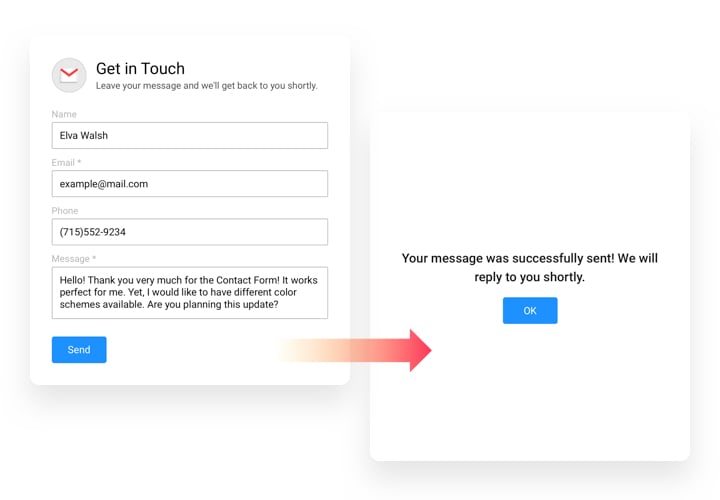The image showcases two pop-up windows designed for customer interaction on a website. 

In the first pop-up window, titled "Get in Touch," there is a form for users to leave their contact information and a message. The form fields include:
- **Name**: Pre-filled with "Elva Walsh."
- **Email**: Placeholder text showing "example at mail.com" with an asterisk indicating a required field.
- **Phone Number**: An empty field.
- **Message**: Contains a pre-written message that reads, "Hello, thank you very much for the contact form. It works perfect for me. Yet I would like to have different color schemes available. Are you planning this update?"

Below the form fields, there is a blue "Send" button with a reddish-orange arrow pointing to the right, inviting the user to submit their message.

In the second pop-up window, a confirmation message is displayed, reading, "Your message was successfully sent. We will reply to you shortly." Beneath this, there is a blue "Okay" button.

The background of these pop-up windows is currently white. The context suggests that this is a demonstration of a contact form interface, likely by a graphic designer, to show its functionality on a website. The customer's message indicates a request for additional color scheme options in future updates.